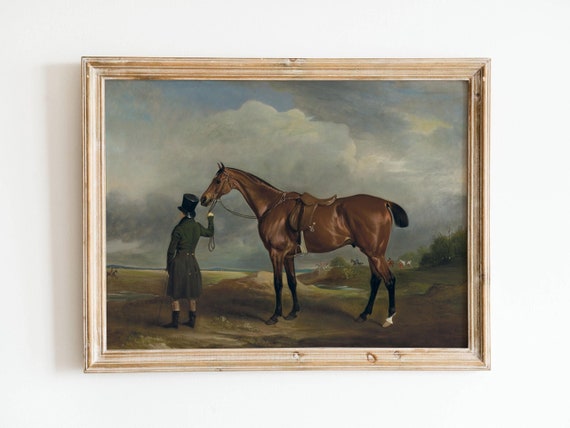This image captures an exquisite painting hanging on a white wall, possibly in a gallery or a home, enclosed within a one-inch light wooden frame that has a vintage, slightly worn appearance. The painting portrays an ambiguous figure, possibly a man or a woman, dressed in an old-fashioned horse riding uniform. This attire includes a black top hat, a long green riding dress or trench coat with a belt, and mid-calf black boots. The figure is leading a majestic chestnut horse, identifiable by its distinctive black legs except for a white spot on its back left hoof, and a short black tail. The surrounding landscape features subtly rolling hills dotted with a few distant horses, trees, and a path along which the figure and the horse seem poised to travel. The sky overhead is predominantly filled with gray clouds, although glimpses of blue sky break through, enhancing the atmospheric depth of the artwork.